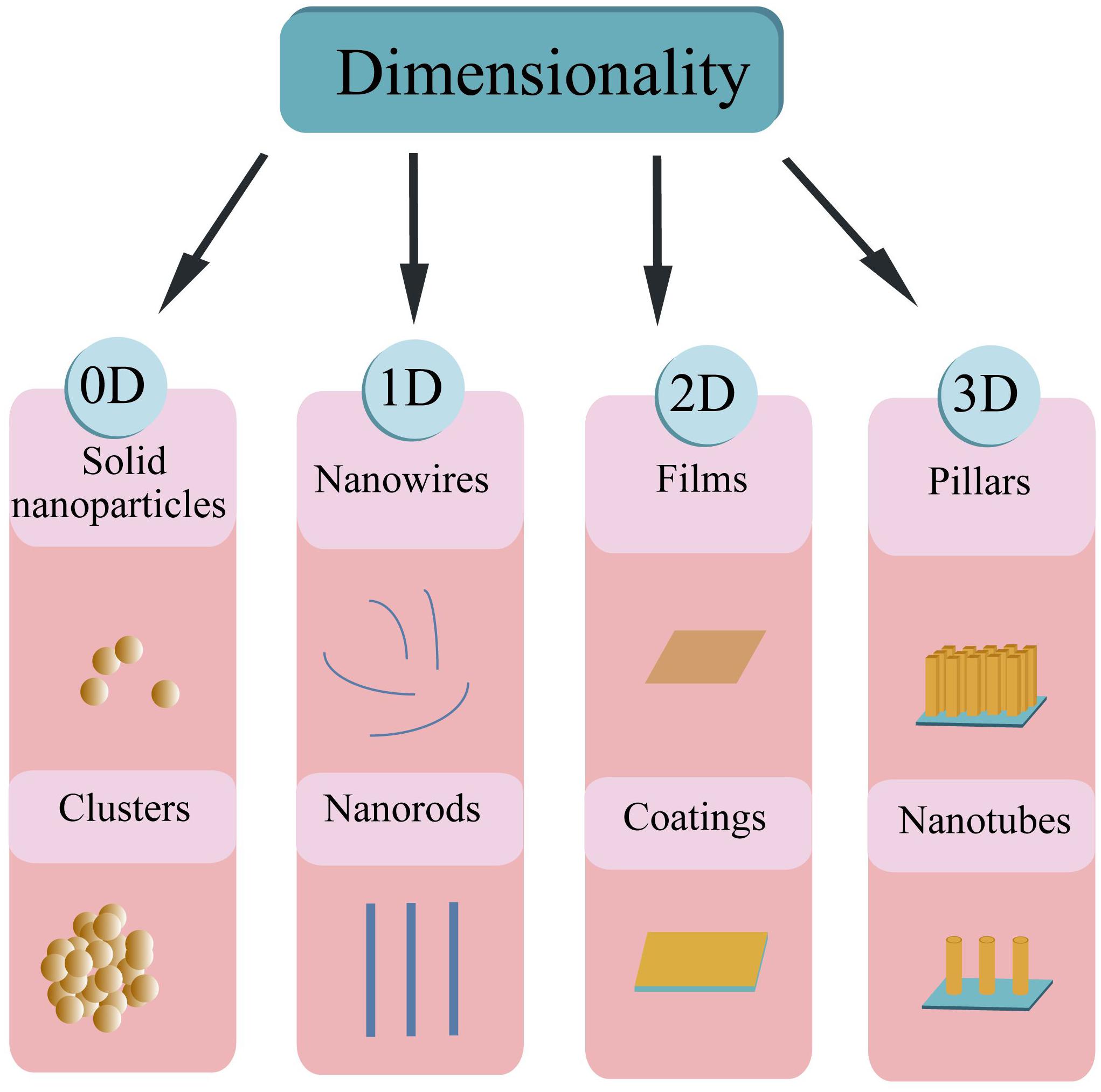The image is a detailed chart titled "Dimensionality" in bold black letters against a blue background at the top. Four black arrows extend downward, pointing to separate sections of the chart that each describe different nanostructures organized by their dimensions. 

The first section on the left is labeled "0D" inside a blue circle. Beneath this, a pink background features descriptions and illustrations: "Solid Nanoparticles" in black text above a pink rectangle containing four grouped round particles labeled "Clusters."

The second section, labeled "1D" also inside a blue circle, includes "Nanowires" with an illustration of four thin lines, followed by "Nanorods," depicted as three slightly thicker rods.

In the central section marked "2D" within a blue circle, it describes "Films" with a tilted gold rectangle on a pink background, followed by "Coatings," illustrated with a similarly tilted, slightly brighter yellow rectangle bordered with blue.

The rightmost section labeled "3D" in a blue circle includes "Pillars," shown as several rods protruding from a blue base, and "Nanotubes," depicted with three larger, separated rods standing on another blue base. Throughout, the visual descriptions are detailed and consistent against the pink background, providing clear examples of each type of nanostructure.